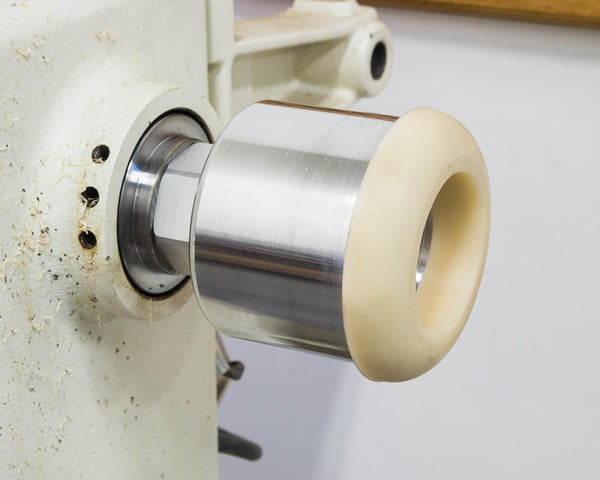The image features an old, rusty door or machine part that appears to be connected to a wood lathe. The centerpiece is a wide, metallic cylinder, possibly a handle or knob, with a rubbery or plastic cream-colored top. This knob is attached to the lathe through a mix of screws, nuts, and bolts. The white surface of the machine it is attached to appears metallic and chipped, showing signs of aging and wear. Surrounding the knob, there are dark holes and some debris, further indicating its old and neglected condition. The area also has old hinges that need cleaning. The background includes a light gray floor and wooden elements, suggesting an indoor setting, possibly a workshop.